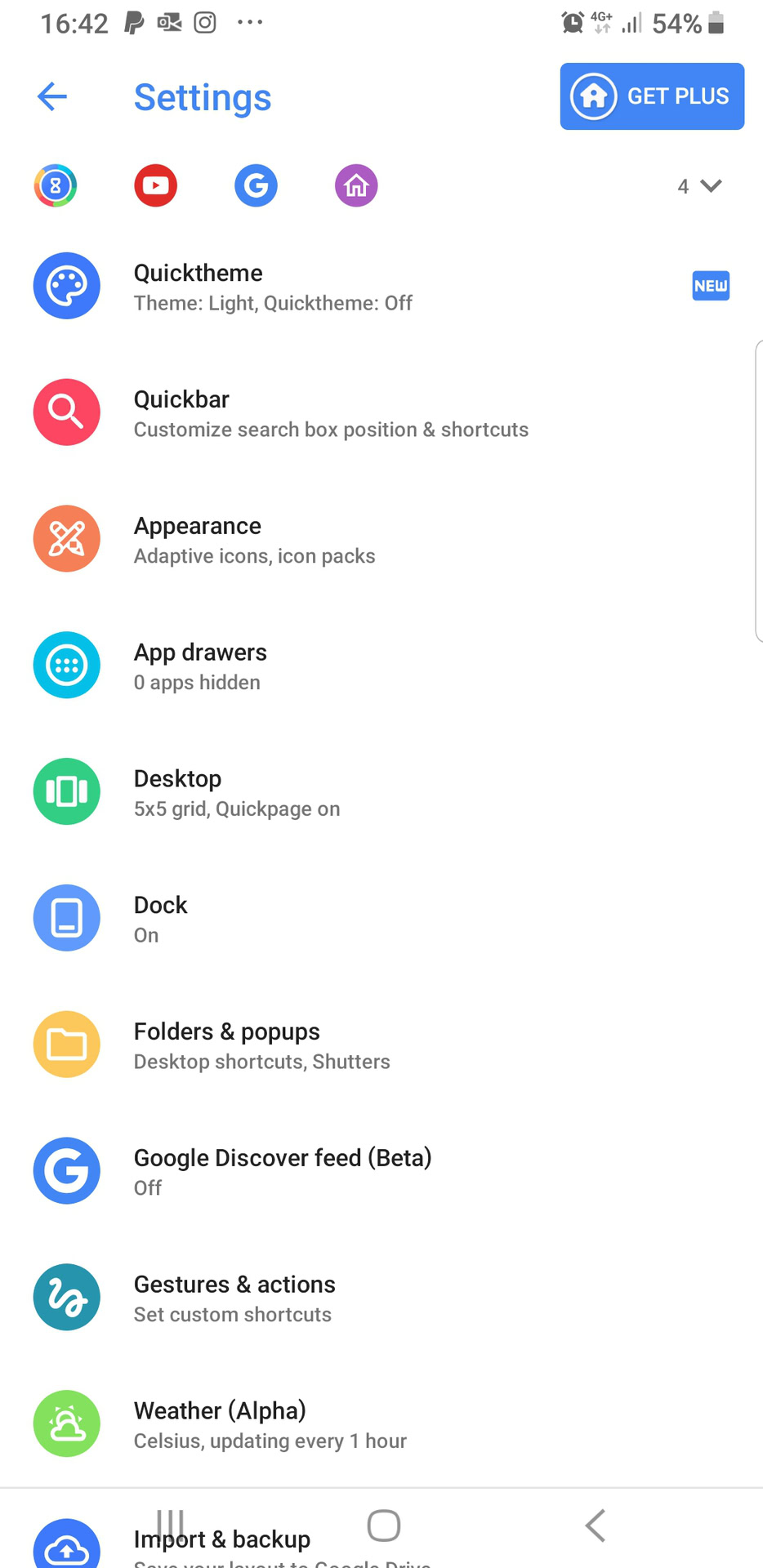A smartphone screen is depicted with a PayPal application open, recognizable by its prominent 'P' logo. To its right, a smaller recording icon is visible, followed by the Instagram app, and a trio of vertical dots indicating additional options. On the upper right corner, the status bar showcases an alarm clock icon, 4G network signal bars, and the battery level indicator. Below these icons is a button labeled "Get Plus" in white text.

In the top left area, there is a house icon enclosed in a circle. Below the main icons, a left-pointing arrow, highlighted in blue, is visible next to a settings icon, also blue. Further down, there are four tiny icons, including an '8' within a circle, YouTube, a 'G' within a circle representing the Google app, and a home icon.

The screen features several more icons and options, including a paintbrush symbol for themes, labeled "Theme Light" and "Quick Theme Off." A red circle with a magnifying glass sits below these options, leading to more selections for appearance, such as app drawers, dock folders, and pop-ups, indicated in orange and blue.

Additional settings include Google Discover Feed (currently off), gestures and actions, and a weather alpha. Further, options for importing and backup are present. At the bottom of the screen, the navigation bar contains three icons: three vertical lines, a square, and a left-pointing arrow.